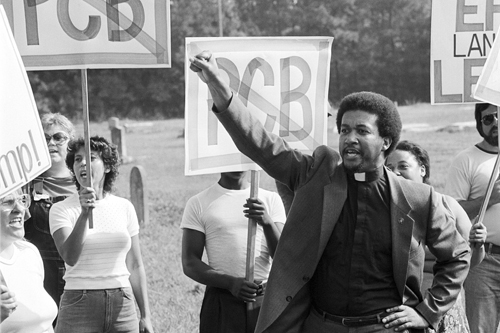This horizontally aligned, rectangular black-and-white photograph, likely taken during the 1960s, depicts a protest scene set outdoors on a grassy area. Central to the image is an African-American man dressed in a priest's attire, identifiable by his black shirt with a white collar and a suit jacket. His short, puffy black hair frames a face caught mid-speech, with his mouth open. He stands with his left hand on his hip, while his right arm is extended upwards in a powerful fist. The background is dense with trees, partially obscured by the square protest signs held by the crowd behind him. These signs prominently feature the acronym "PCB," although the exact meaning remains unclear. The diversity of the protestors suggests a varied racial composition, adding to the gravity and historical significance of the demonstration.